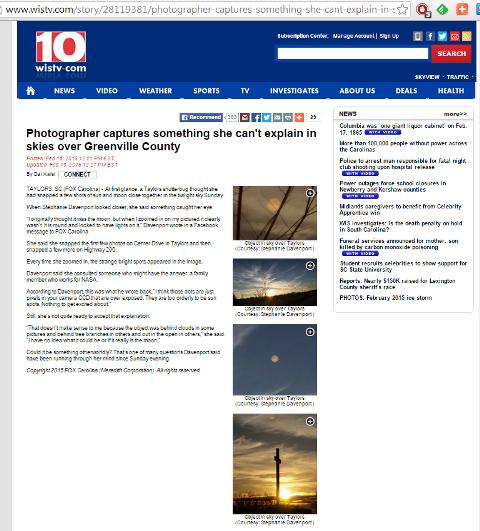This screenshot from the news website www.wistv.com displays a detailed webpage layout, featuring both site navigation elements and a visually compelling news story. At the very top, the web address is clearly visible, and to the right, several icons provide additional functionalities. The page navigation includes a striking blue box featuring the station's logo, a tin icon, and a red box with a white outline, marked with "wistv.com." Adjacent to this, there is a search bar with an elongated, blank entry field and a Search button, set against a red background with white text.

The main content of the webpage features a prominently displayed news story titled, "Photographer Captures Something She Can't Explain in Skies Over Greenfield County." Below the headline, the publication time of the article is noted in smaller red text, while the body of the story appears in standard black text, providing a readable contrast.

Accompanying the article are four evocative photographs related to the story, arranged vertically. The first image depicts a sky with a brownish-gray hue, framed by tree silhouettes in the foreground. The second image captures a picturesque sunrise, with wispy white clouds and a brilliant blue sky, and a stunning red horizon illuminated by the rising sun. The third photo shows a mysterious round circle in a bluish-gray sky, enhanced by wispy clouds. The final image presents a cross-shaped form amidst a cloudy sky, with the sun peeking over the horizon.

On the right side, a section labeled "News" provides links to additional news stories, enriching the webpage with more content for the reader's exploration.